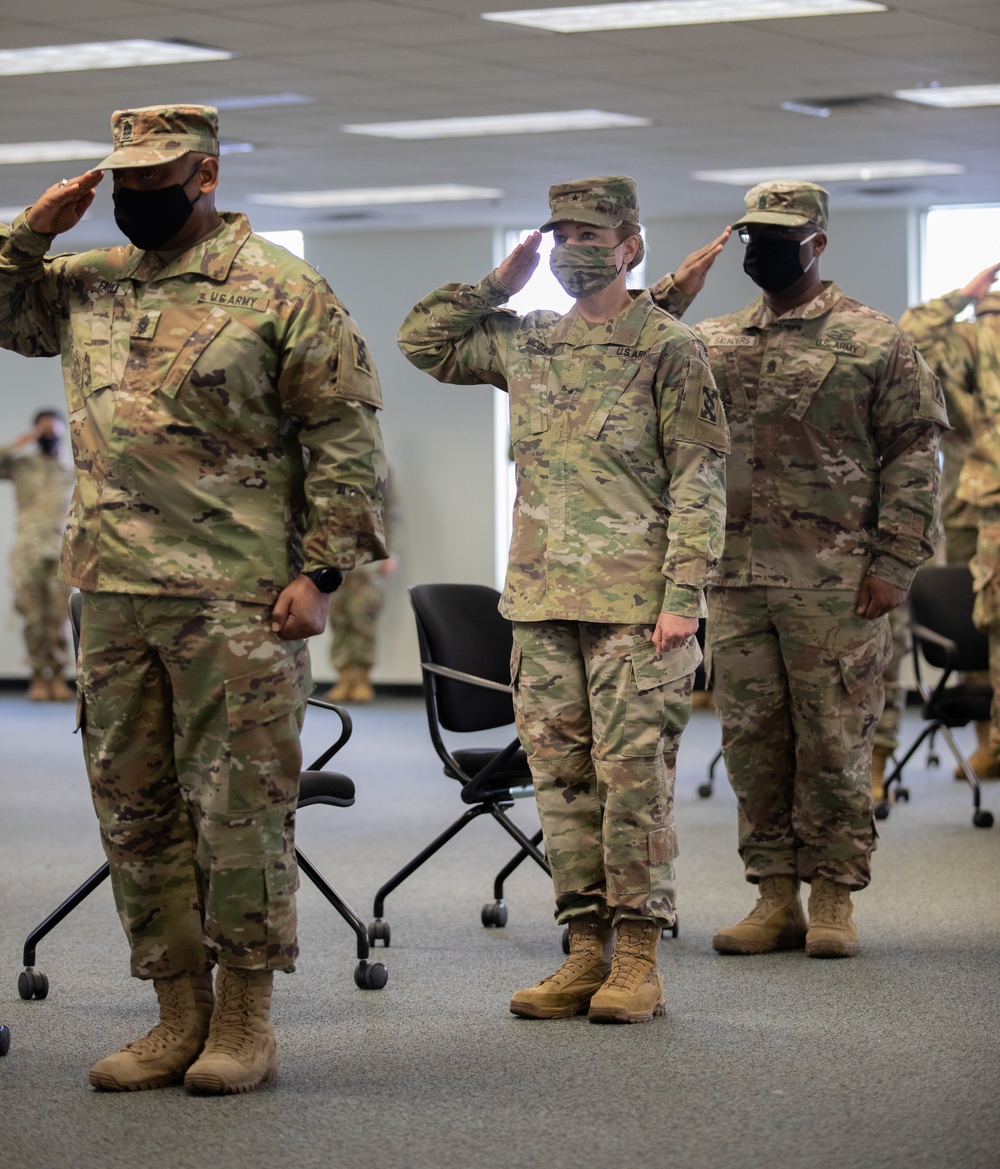In this image, a group of soldiers stands in a lined formation inside a brightly lit office setting. Each soldier is dressed in full camouflage uniform, including matching hats and black face masks, except for a female soldier in the middle wearing a camouflaged mask. They all wear tan boots and salute solemnly, appearing to have just stood up from the black rolling desk chairs behind them. The gray carpeted floor and white walls of the room complement the scene, which is framed by additional soldiers in the background who are also saluting in unison. The chairs and the neat alignment of the soldiers suggest a formal occasion or ceremony.